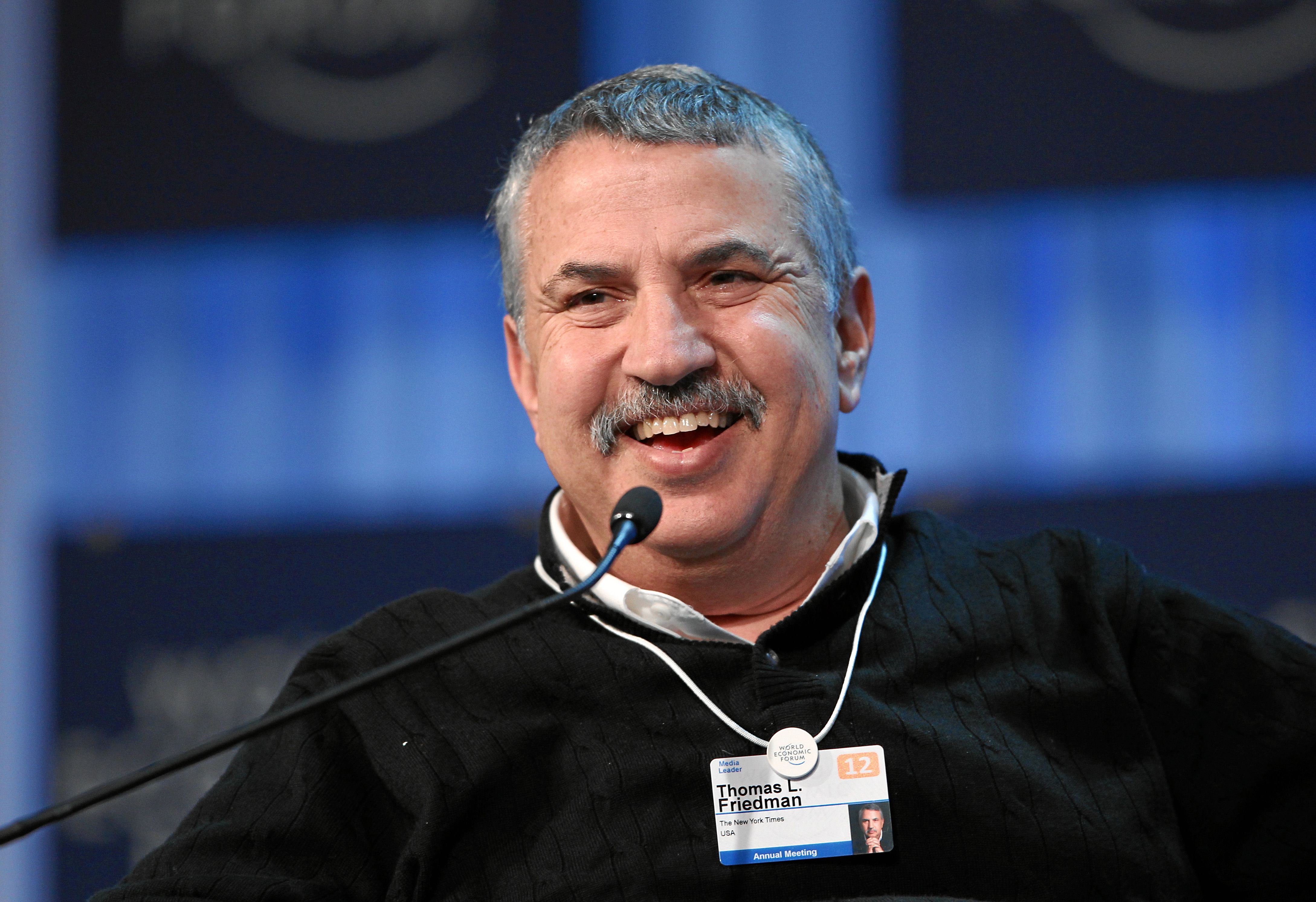The photograph captures Thomas L. Friedman, identifiable by the name tag hanging around his neck, which has his photograph and the text "Thomas L. Friedman" in black, and a number "12" in white and yellow. He appears to be seated, likely at a conference, as suggested by the microphone positioned in front of him on a stand. Friedman is wearing a dark sweater—possibly black or dark brown—with intricate cable knitwork over a white, open-collared undershirt. He has short, mostly gray hair with darker tones on top, along with a matching blackish-gray mustache and dark eyebrows. He's slightly overweight, with a cheerful expression, smiling or about to speak into the microphone. The background, although out of focus, features shades of blue and black, and possibly red squares, hinting at a large venue or stage setting.